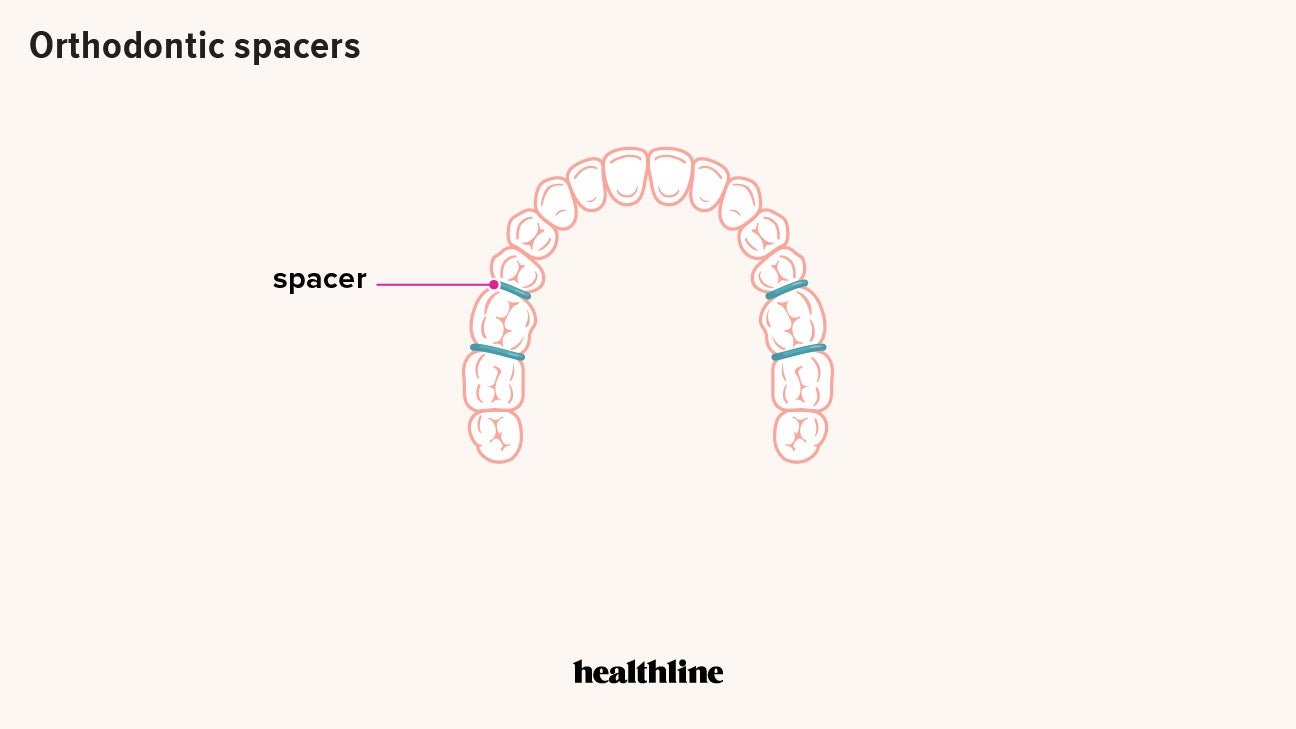The image is a straightforward, clipart-style diagram illustrating orthodontic spacers. The background is light beige, and it features an overhead view of a row of teeth, likely the lower jaw, outlined in orange. The title "Orthodontic Spacers" is prominently displayed in black font at the top left corner. The diagram shows green lines, identified as spacers, placed between some of the molars towards the back of the mouth, with one red line pointing to a green spacer for emphasis. The image is minimal in color and detail, focusing instead on clearly depicting the spacers' placement and function. A caption at the bottom center reads "Healthline," indicating the source of the image.